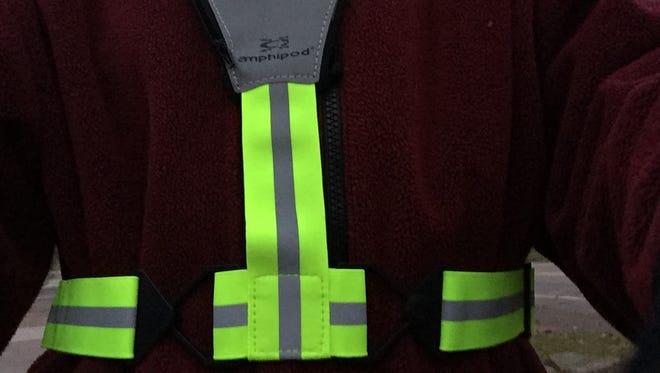This up-close photograph showcases an individual dressed in a dark brown, baggy, utility jumpsuit, prominently featuring safety gear designed for visibility. Neon yellow-green reflective straps are strategically positioned, with one vertical strap running down the center of the torso and a horizontal strap circling the waist. These bright, fluorescent straps ensure visibility in low-light environments. Attached to the upper middle of the vertical strap, a gray piece bears the brand name “Amphipod" in lowercase letters, marked by a small frog logo. Behind the individual, glimpses of a gravel-strewn street and dirt can be seen. The jumpsuit itself is notably loose, with fabric bunching up, highlighting the functional, rugged design of the attire.